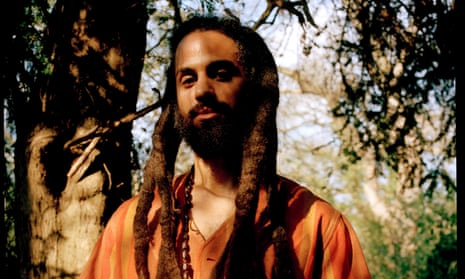This photograph captures a man standing in a wooded area on a clear, blue-skied day. The image focuses on him from the chest up, emphasizing his thick brown dreadlocks, brown beard, and slightly shadowed face. He wears a distinctive, orange V-neck shirt made of a silky material, with the V slightly revealing his chest. His expression appears neutral as he looks directly at the camera. To his left, a thick tree trunk, varying in shades from light to dark brown, occupies about a quarter of the frame. The trunk and the foliage behind cast shadows, blending into the warm golden tones that blanket the background. On his right, the silhouette of a leafy tree is visible. The overall scene, filled with layers of tree limbs and leaves, creates a serene and natural setting, with no additional elements to distract from the vibrant, earthy ambiance.